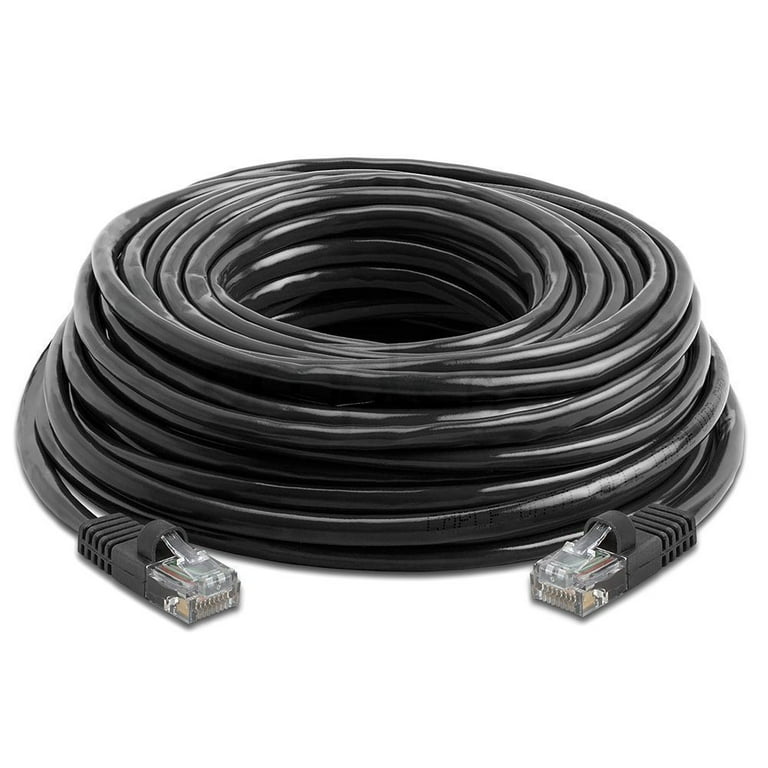The image depicts a coiled 50-foot length of black Cat 5e Ethernet cable, neatly looped and standing upright, forming a round spool with a large hollow center. The cable features high-quality, glossy black sheathing and ends in clear, molded male connectors with gold connector pieces. Designed with strain reliefs, the connectors are fitted with clear protective release tongs to prevent accidental pressing. The cable's functionality is ensured by its robust design, suitable for connecting to routers, computers, or modems.